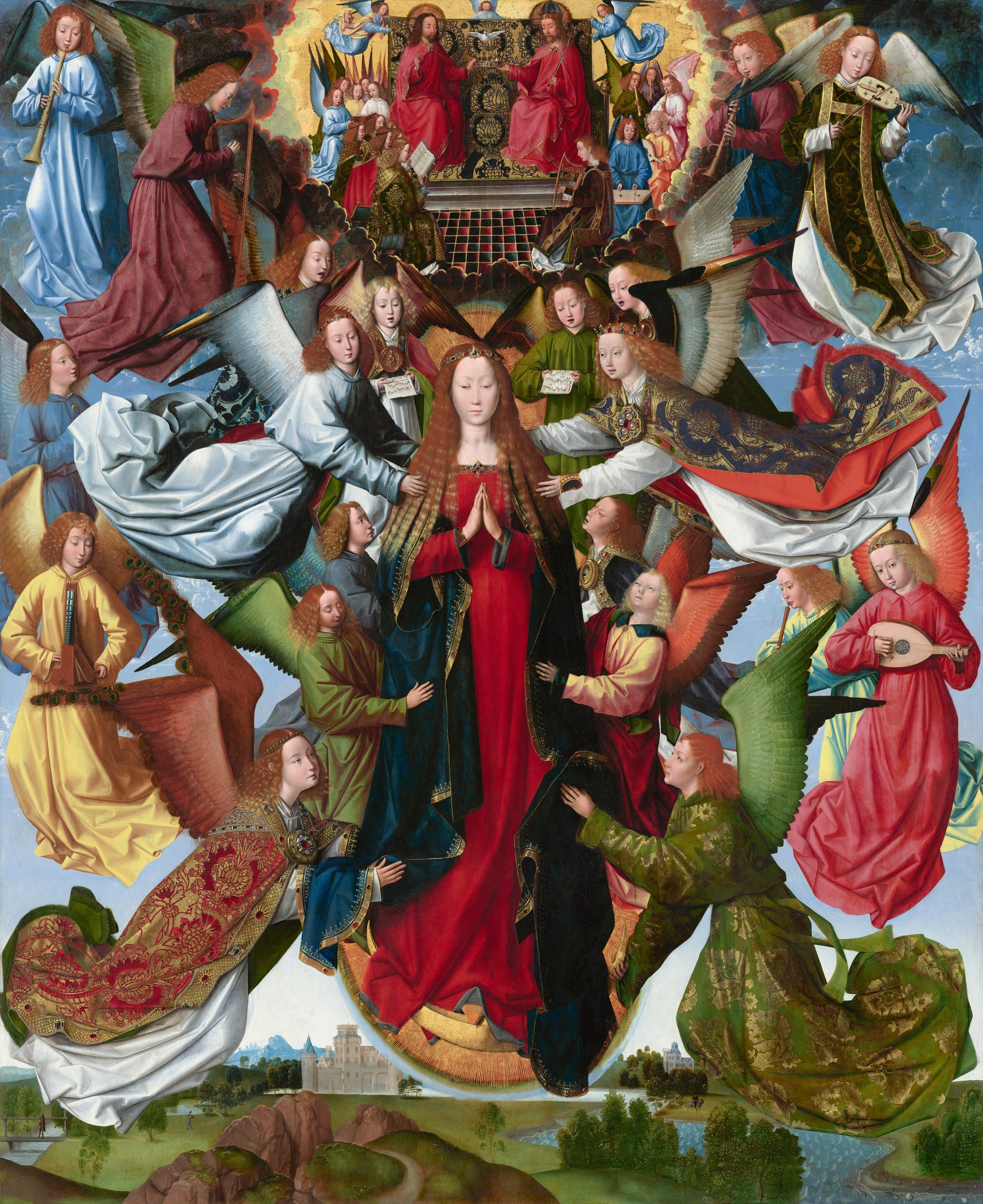The image depicts a central figure, Mary, the queen, standing tall in a long red dress with a green robe draped over her shoulders. She has long brown hair, pale skin, and a small crown atop her head. Her hands are held together in a praying posture at her chest. Surrounding Mary are numerous female angels with wings of various colors—white, green, brown, blue, red, and yellow. The angels, adorned in vibrant garments that match their wing colors, seem to be engaging in musical activities, playing instruments like lyres and flutes, and some are holding up parts of Mary's robe. In the background, a serene blue sky stretches across while beneath, there is a village scene with a river to the bottom left and a gray building in the far distance. The scene appears lively and ornate, with the angels floating and creating a sense of heavenly harmony around the central figure of Mary. The bottom right shows the angels clutching the lower part of Mary's robe with one of the prominent angels having green wings and attire. The image carries the aesthetic of an old-style painting or perhaps a computer-generated image, rich with color and detail, suggestive of a Roman empire-like backdrop.